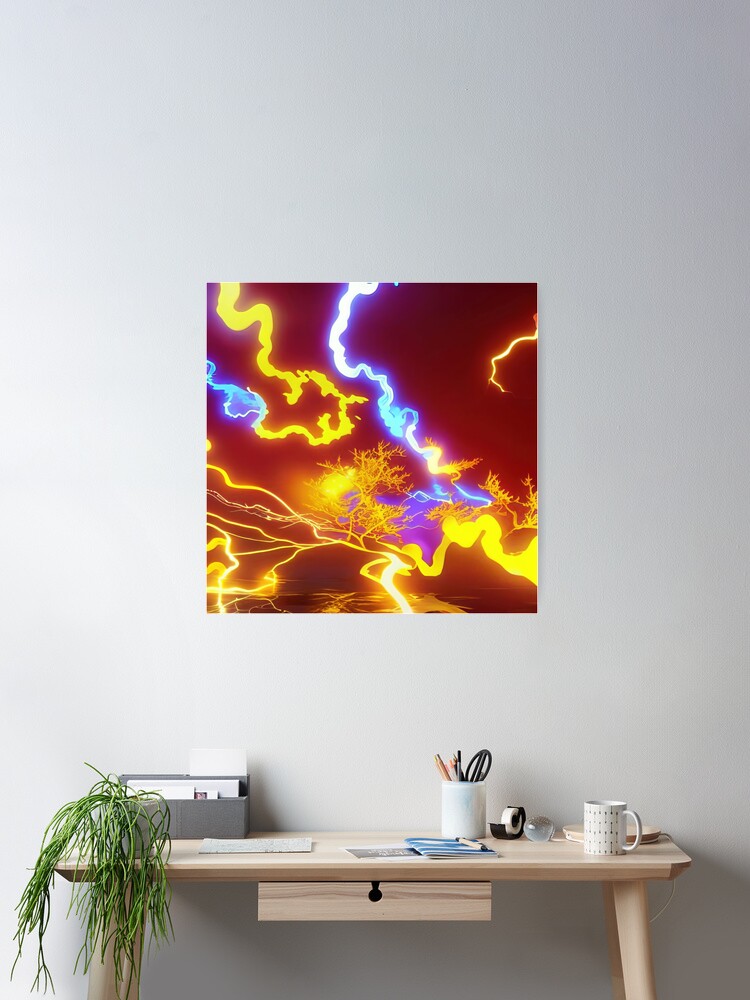A detailed image depicts a white-gray wall as the backdrop, adorned with a striking square poster. The poster features vibrant, yellow lightning bolts radiating from the center towards the bottom left and right corners, with some bolts extending to the top left and top right. A character with a blue outline appears to be skating across these bolts. Below the figure, additional blue lightning bolts cascade downward. 

The scene also showcases a pale brown wooden table with one central drawer. The table supports a variety of items: a weepy-looking green plant in the bottom left corner, a sleek modern white reading lamp on the right, and a white coffee mug. There’s also a gray box with stationary supplies, blue colored paper, a white sheet of paper, and a small pencil holder filled with pens, pencils, scissors, and a roll of tape. The composition includes plenty of negative space, accentuating the vivid artwork and meticulously arranged desk items.